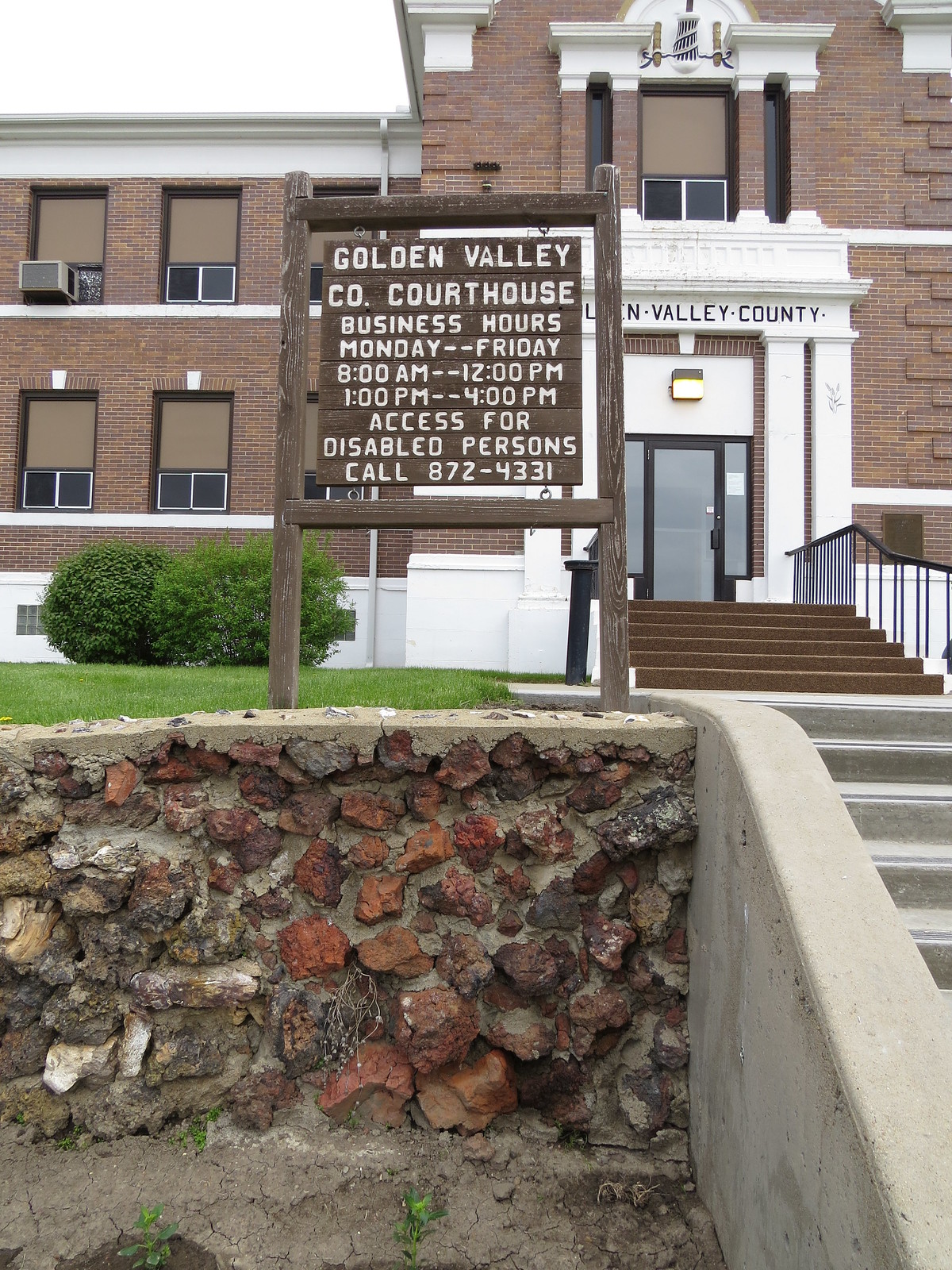The photograph captures the view in front of the Golden Valley County Courthouse. Central to the image is a square, brown painted wooden signpost, from which a wooden plank sign hangs by four circular mounts. The sign, painted with white lettering, announces the "Golden Valley Co. Courthouse" and details the business hours as Monday to Friday, 8am to 12pm, and 1pm to 4pm, also providing a contact number, 872-4331, for disabled access. To the right of the sign is a set of concrete stairs leading to the main entrance of the building. To the left and beneath the sign, a retaining wall constructed from various red and brown stones in concrete is visible. The courthouse itself is a tall, imposing two-story structure made of red brick and accented with white stone trim and white columns. Above the entrance, which features a glass door flanked by glass windows, the words "Valley County" are inscribed on a white awning.